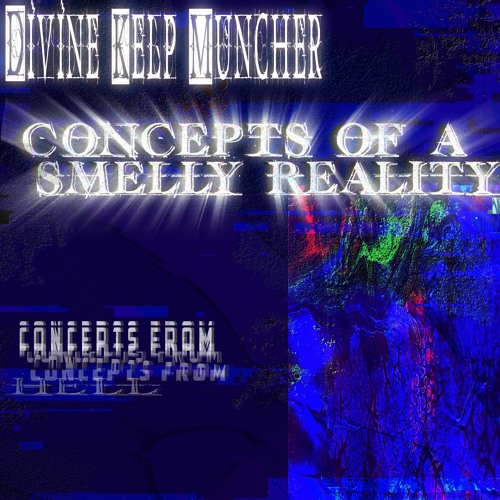This digital image, possibly an artwork, title page of a music CD, or an advertisement, predominantly features shades of blue with occasional swirls of neon pink and neon green on the right side. The abstract design on this side adds an eclectic and dynamic feel, resembling distorted static on a TV screen. Central to the image is glowing white text with bursts emanating from each letter, enhancing its radiant effect. The main captions read: "Divine Kelp Muncher," "Concepts of a Smelly Reality," and "Concerts from Hell." The stark contrast between the deep dark blue background and the intense white lettering, along with occasional oil-like streaks of green and red, creates a visually striking and somewhat chaotic composition. This vivid imagery and text suggest themes of surrealism and intensity, likely tied to the unconventional nature of the advertised content.